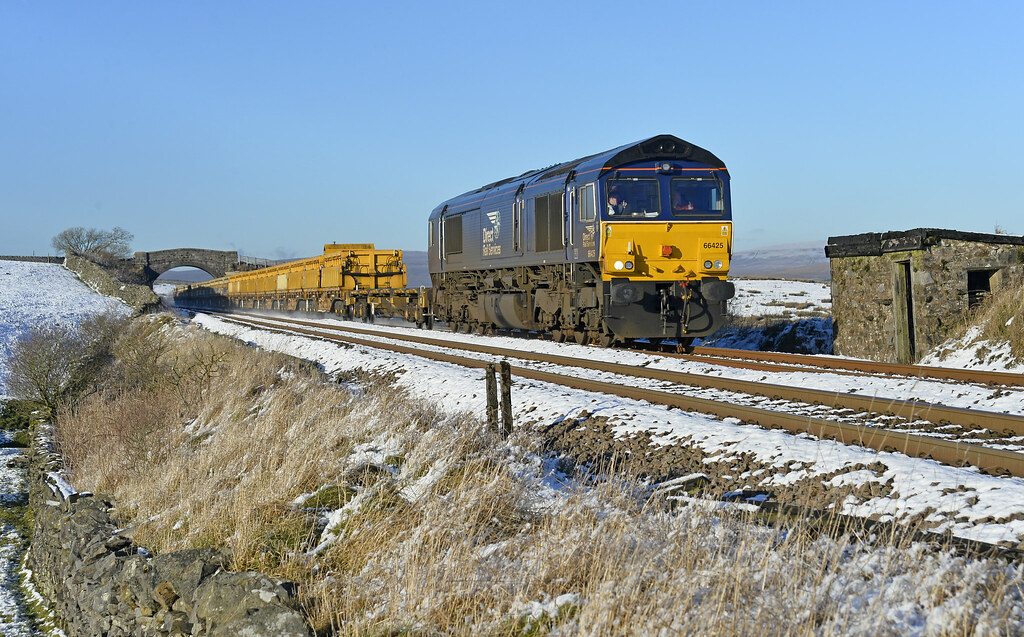This photograph captures a striking landscape featuring a train amidst a serene scene. The top half of the image is dominated by a light blue sky that sets a calm backdrop. In the distance, gently sloping, fairly flat hills appear slightly blurry, enhancing the sense of depth.

The train tracks, rust-colored and running diagonally across the frame, lead the eye upwards to the left. Near the horizon, there is a thin-arched, stone bridge, likely a road crossing over the tracks, adding an element of architectural interest.

The train itself, positioned towards the right of the image, boasts a bright yellow bottom transitioning to blue at the top, with additional blue sides. Behind the locomotive are several train cars, primarily yellow in color. This vibrant train contrasts sharply against the muted tones of the landscape.

Surrounding the tracks, a light dusting of snow covers the ground, noticeably absent from the tracks themselves. Dry brown grasses and a gravel bed characterize the hill leading up to the tracks, with small patches of green ground peeking through. Beige reeds and partially melted snow patches add texture to the scene.

Adding a quaint touch, a little stone hut sits to the right of the train, completing this picturesque and tranquil vista.